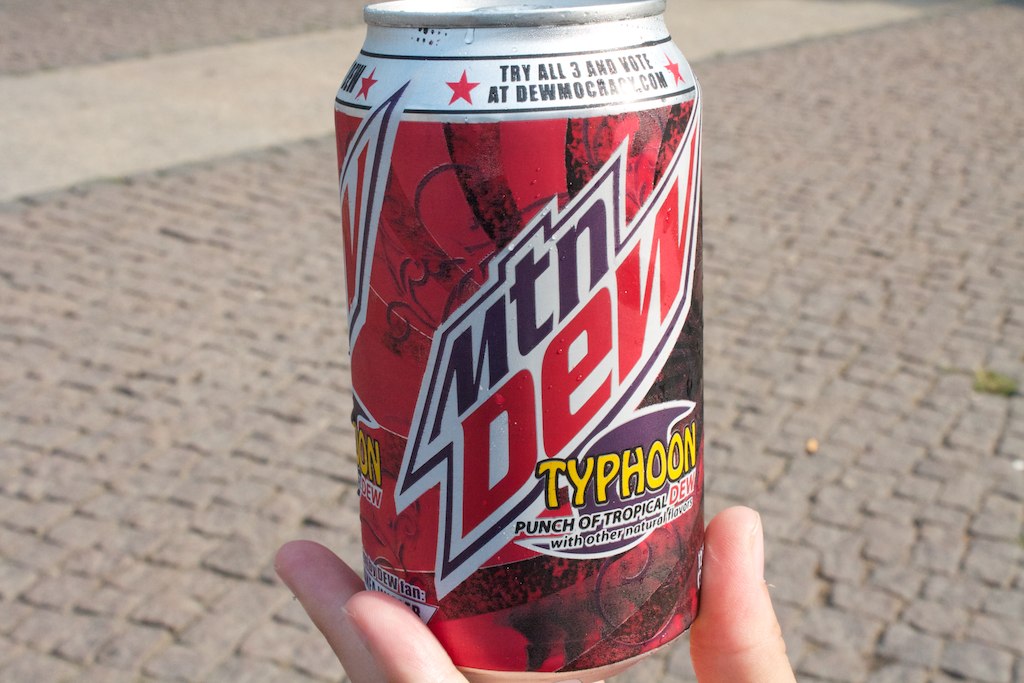A vivid rectangular photograph in landscape orientation captures a person's left hand holding a can of Mountain Dew Typhoon Punch. The can stands out with its striking design: a silver base adorned with a dynamic red and black background. The iconic "Mountain" is printed in bold black lettering, while the "Dew" is vividly highlighted in red. The word "Typhoon" is prominently displayed in bright yellow, emphasizing the tropical flavor of the drink. The hand holding the can is delicately positioned, indicating careful grip and focus on the product. The backdrop complements the subject with a light gray cobblestone ground, adding a subtle yet textured contrast to the bold colors of the can.